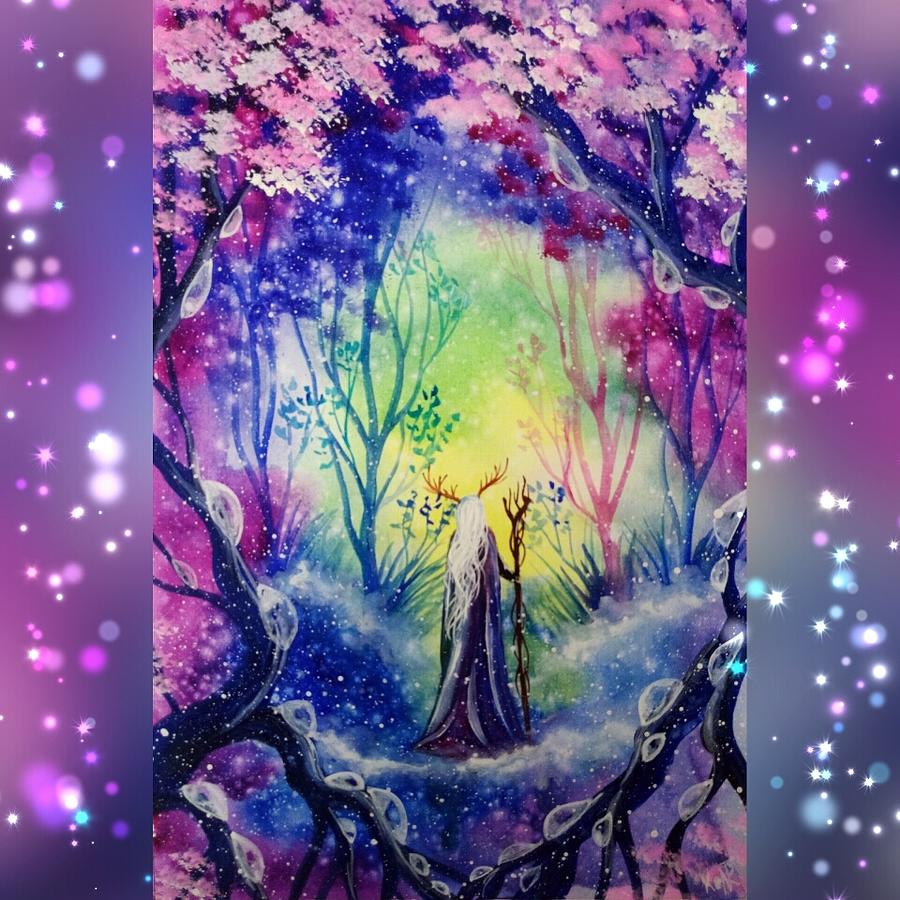In this captivating digitally generated illustration, a figure stands at the heart of a fantastical forest. This humanoid, possibly a wizard or elf, is clad in a flowing purple cloak with white streaks and possesses long white hair cascading down to the middle of their back. They grasp a wooden staff in their right hand, and red antlers protrude from their head, adding to their mystical aura. The enchanting forest surrounding them is adorned with trees in hues of gray, green, pink, and blue, while pink and red flowers and lush green leaves and grass carpet the forest floor. White flecks resembling falling snow and a starry, pink sky add a celestial touch to the background. The scene is bathed in a soft yellow glow at its center, casting an ethereal light over the enchanting woodland.